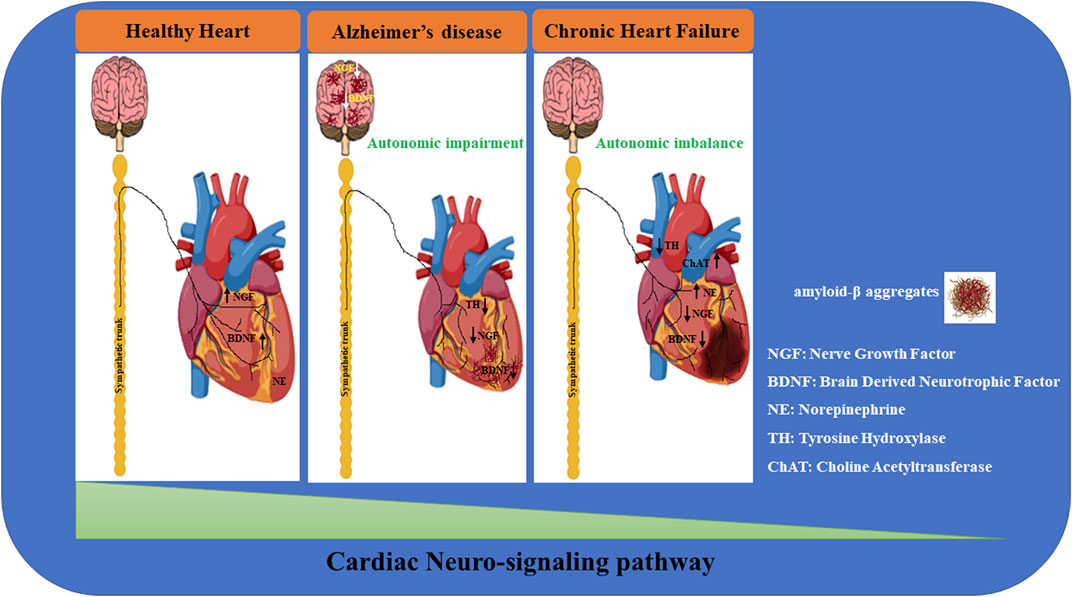This educational image provides a detailed depiction of cardiac neuro-signaling pathways on a blue background and is rectangular with curved corners. The left side features three white-background sections, each containing a diagram showing the heart, brain, and sympathetic trunk spinal cord. The first section, titled "Healthy Heart," shows normal connections, including arrows indicating NGF to a blue vessel and BDNF to a neural attachment. The second section, labeled "Alzheimer's Disease," illustrates autonomic impairment with downward arrows for TH and NGF, indicating issues like disconnection. The third section, titled "Chronic Heart Failure," highlights autonomic imbalance with downward arrows for TH, NGF, and BDNF, and upward arrows for CHAT and NE, showing a significantly darkened problematic area on the heart's lower right. The right side of the image features white text listing key neurological and biochemical factors: amyloid-β aggregates, nerve growth factor (NGF), brain-derived neurotrophic factor (BDNF), norepinephrine (NE), tyrosine hydroxylase (TH), and choline acetyltransferase (CHAT). At the bottom center, red and black text reads "Cardiac Neuro-signaling Pathway."